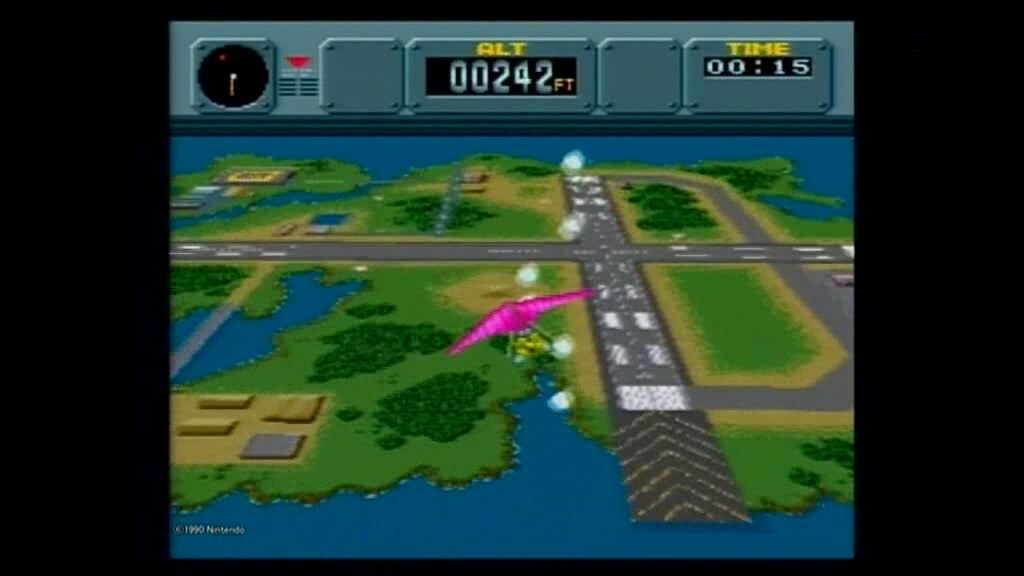This color image is a pixel art screenshot from an old video game, resembling titles that might have been on the NES or Sega systems. The user interface at the top of the screen resembles an instrument panel with a metallic design. In the top left, there's a clock that might be a radar or compass, flanked by artistic vent-like features and an empty panel. In the center, a yellow label reads "ALT" with the number 0042 below it, indicating the altitude. On the right, another yellow label says "TIME" with a timer displaying 00:15.

The main image shows a scene of someone in a pink hang glider soaring over an island, which features an airport runway amid green trees and some brown patches. The person under the glider appears to be wearing yellow. There are small buildings visible on the left side of the island, indicating a simple, yet detailed overworld typical of vintage video games.